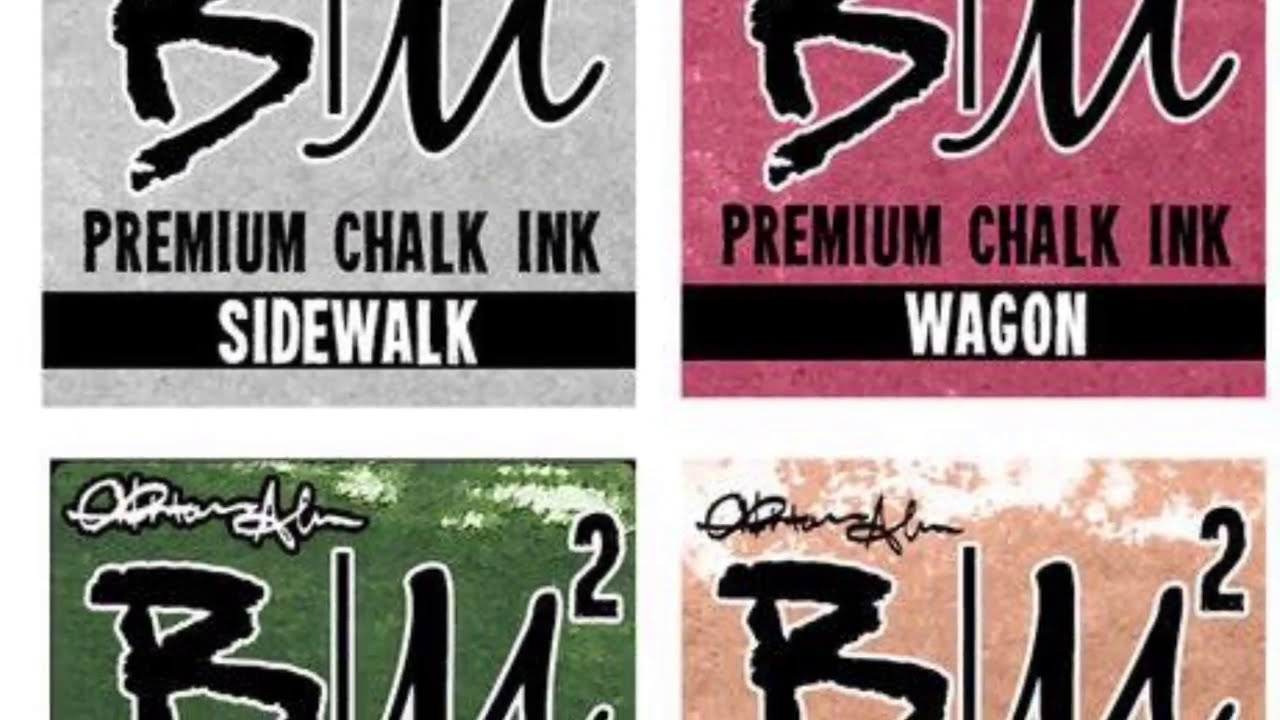This image is divided into four quadrants, each displaying a different colored background and partially visible text. In the upper left quadrant, set against a gray background, the text reads "BLM" followed by "Premium Chalk Ink" and then "Sidewalk." The upper right quadrant features a reddish-pink background with the same initial text "BLM" and "Premium Chalk Ink" but ends with the word "Wagon." The bottom halves of both the lower left and lower right quadrants are cut off, obscuring the full text, though the visible parts indicate a similar layout. The lower left quadrant has a dark green background and the lower right has a tan or peach background, each still displaying the letters "BLM." Additionally, each quadrant appears to feature a signature or a number two in the upper left corner. The image as a whole seems to be an advertisement for different colored varieties of premium chalk ink.